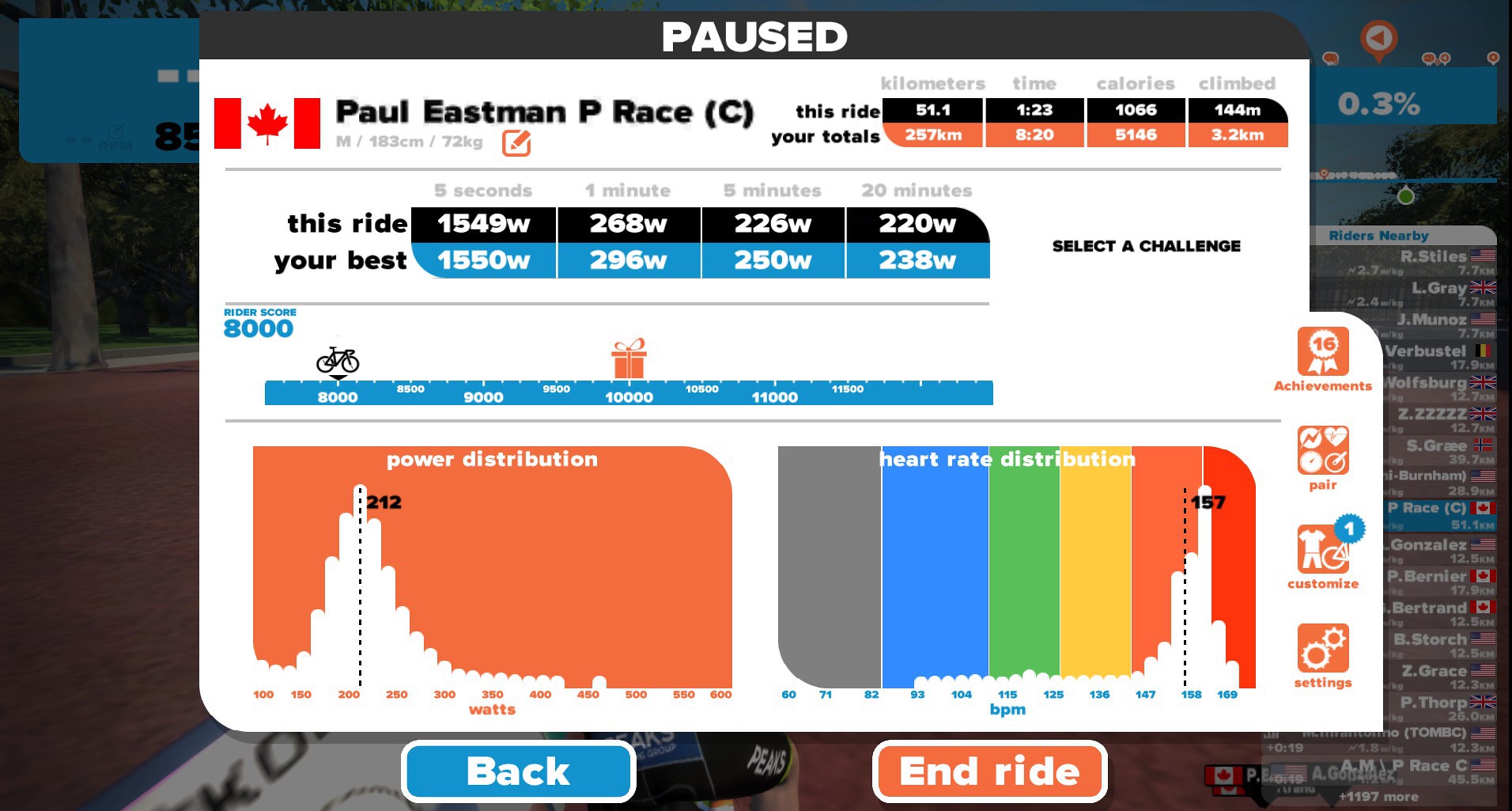This horizontally aligned rectangular image appears to be a screenshot from a high-tech, gamified exercise bike interface, designed to track and display detailed rider statistics. At the top, a grey bar spans the width of the screen, featuring the word "PAUSED" in white text. To the left of this bar is a Canadian flag icon, followed by the name "Paul Eastman P. Race (C.)". Below this is a white rectangular section providing a summary of the current ride, with statistics including: distance (51.1 kilometers), elapsed time (1 minute and 23 seconds), calories burned (1066), and elevation climbed (144 meters).

Further down, there are segmented graphs categorizing time intervals of 5 seconds, 1 minute, 5 minutes, and 20 minutes, comparing the current ride to personal bests. Below these data points, there are two additional bar graphs displaying "Power Distribution" against an orange background and "Heart Rate Distribution" with various colors. The layout also includes navigational buttons at the bottom: "Back" in white text on a blue background under the power distribution graph, and "End Ride" in white text on an orange background under the heart rate distribution graph. On the sides of the image, parts of a virtual road and track interface are visible, suggesting the context of a racing game or virtual ride, where other users and their information are displayed.